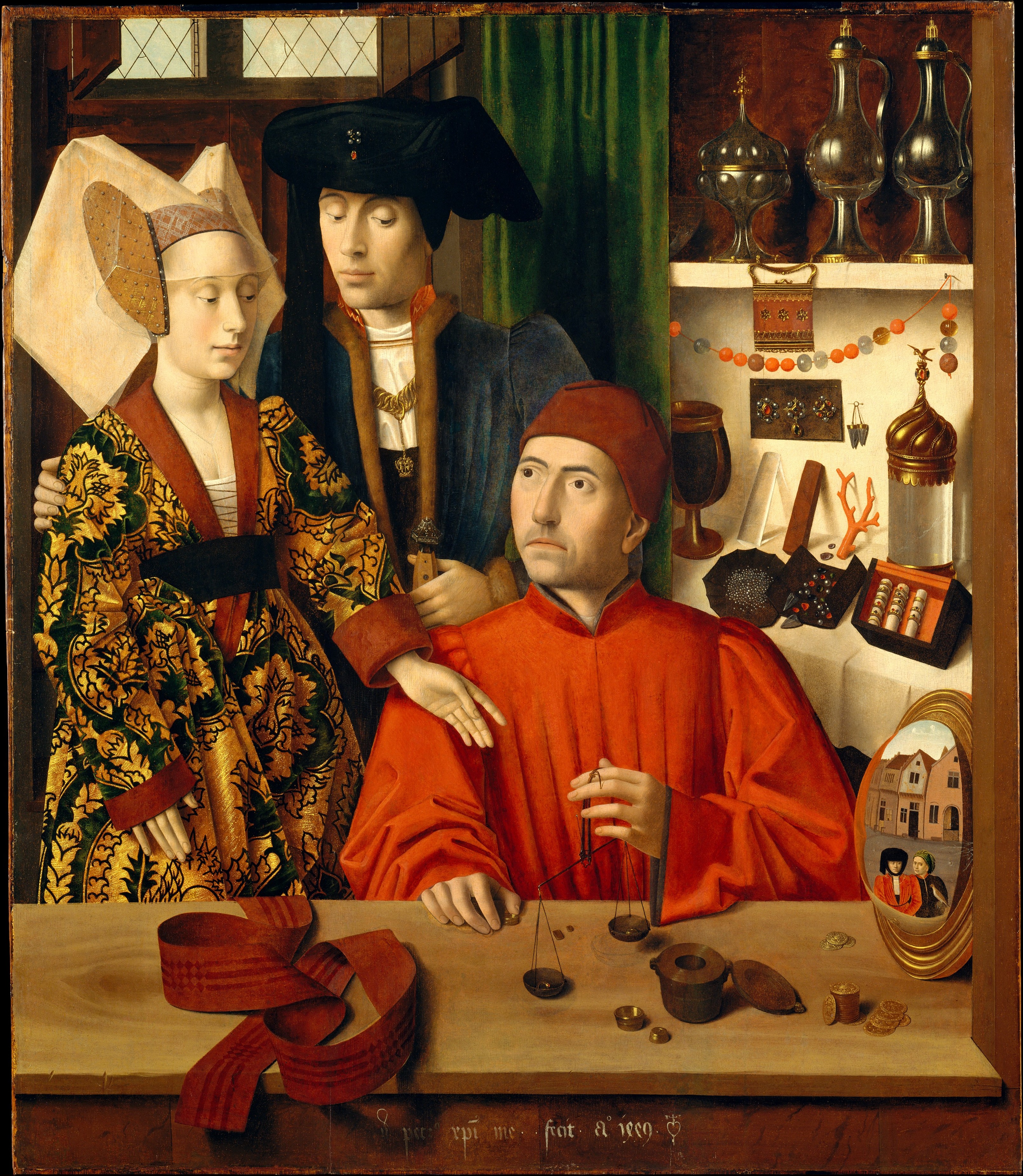This painting, reminiscent of the Renaissance era, captures an intricate scene involving three figures dressed in elaborate, period-specific attire. At the center, a man sits at a brown wooden desk, adorned in a long-sleeved orange robe and matching cap. His contemplative gaze is directed off into the distance as he steadies a pair of scales with his hands. Around the desk, various items such as weights, a red ribbon, and a photo are subtly detailed.

Behind him, slightly over his shoulders, stands a woman and a man. The woman is donned in a vividly ornate tunic dress with a predominant yellow-green satin fabric, intricately trimmed with red, and accented with a black belt around her bodice. Her look is completed with a peculiar headdress. She appears to be extending her left hand towards the seated man as if expecting something in return. On her shoulder, the man standing next to her seems protective, his eyes subtly fixed on the man at the desk. He wears a blue velvet robe, coupled with a stylish black hat, a white shirt, and a distinguishable gold medallion.

The backdrop completes the scene with a window flanked by green drapery and wooden paneling. Shelves brimming with bottles, glasses, pieces of artwork, and trinkets subtly intensify the historical ambiance of the room, enriching the overall depiction of this Renaissance tableau.